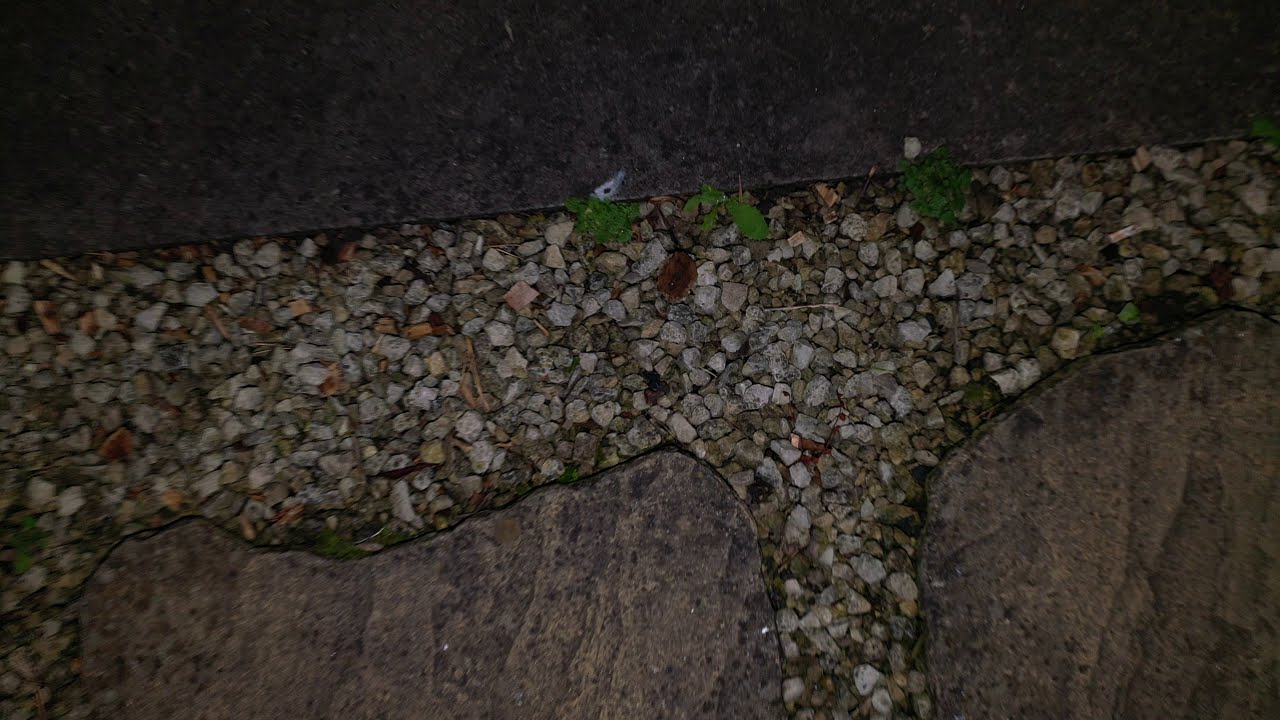The image showcases a section of a stone walkway, possibly leading to a house. Dominating the scene are large, naturally shaped gray paving stones, with concave and convex edges, exhibiting a range of colors from beige to dark gray. These pavers are interspersed with small, white pebbles, which are mixed with shades of black and various beiges, creating a textured and varied appearance. Sparse green weeds are seen sprouting through the pebbles, adding a touch of organic life to the scene. A solid, straight-line concrete border neatly frames the entire area, giving structure to the otherwise natural layout. The surface appears wet, suggesting a recent rainfall, which enhances the vividness of the stones and pebbles. The close-up perspective emphasizes the intricate details and textures of the stones, pebbles, and emerging greenery.